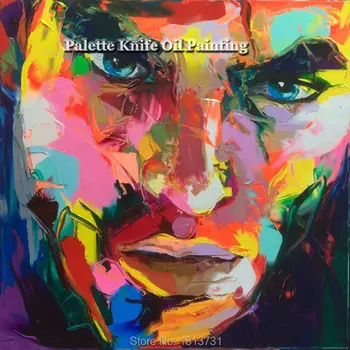The image is a vibrant and abstract close-up of a man's face, rendered in a palette knife oil painting style. The artwork features a myriad of bright colors, including pink, blue, yellow, red, and orange, creating a striking and colorful composition. The man has distinct blue eyes and heavyset black eyebrows, with his face visible from his forehead down to the bottom of his chin. The eyes are positioned slightly above the center of the image. The background, visible around the sides of his chin, includes darker hues combined with purple, green, and orange. Across the left eye of the painting, white text reading "palette knife oil painting" stretches from the left side of the left eye to the left side of the right eye. At the bottom, underneath the man's chin, semi-transparent white text reads "store," followed by a sequence of numbers that are difficult to discern. A shadowy region appears in the bottom right-hand corner of the image. Overall, the painting is vibrant, clear, and high-quality, showcasing a blend of detailed facial features and abstract color combinations.